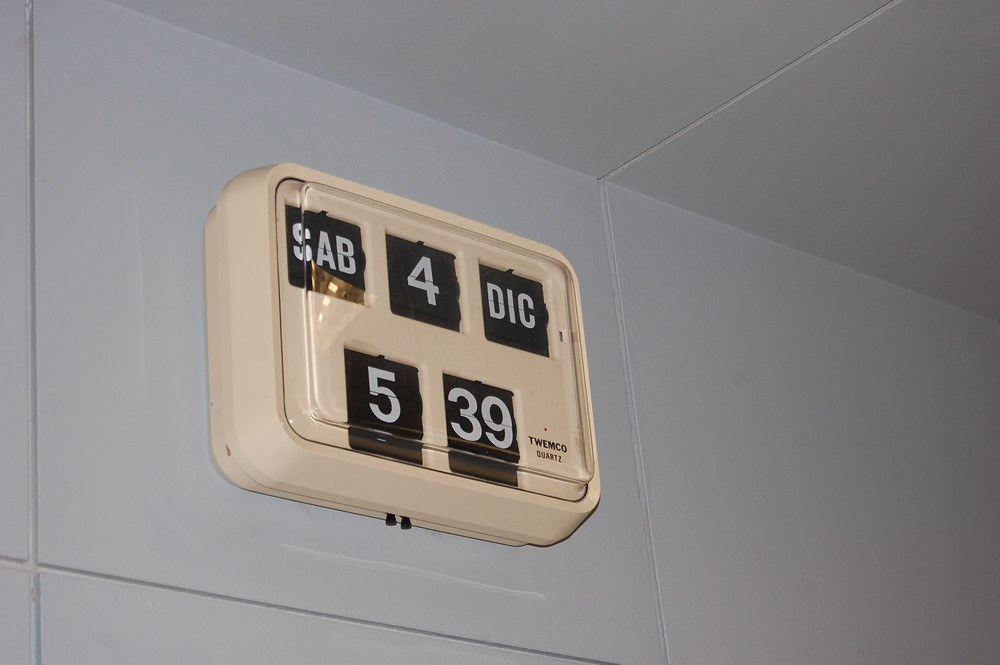A vintage analog clock is prominently displayed against a stark white wall. The clock, with its beige casing and classic design, features a black face with white text displaying the time as 5:39. The date indication on the clock reads "sab" and "deke," suggesting that the language is not English. The simplicity of the clock and the unadorned, plain white backdrop highlight the clock’s old-fashioned charm and functional elegance.